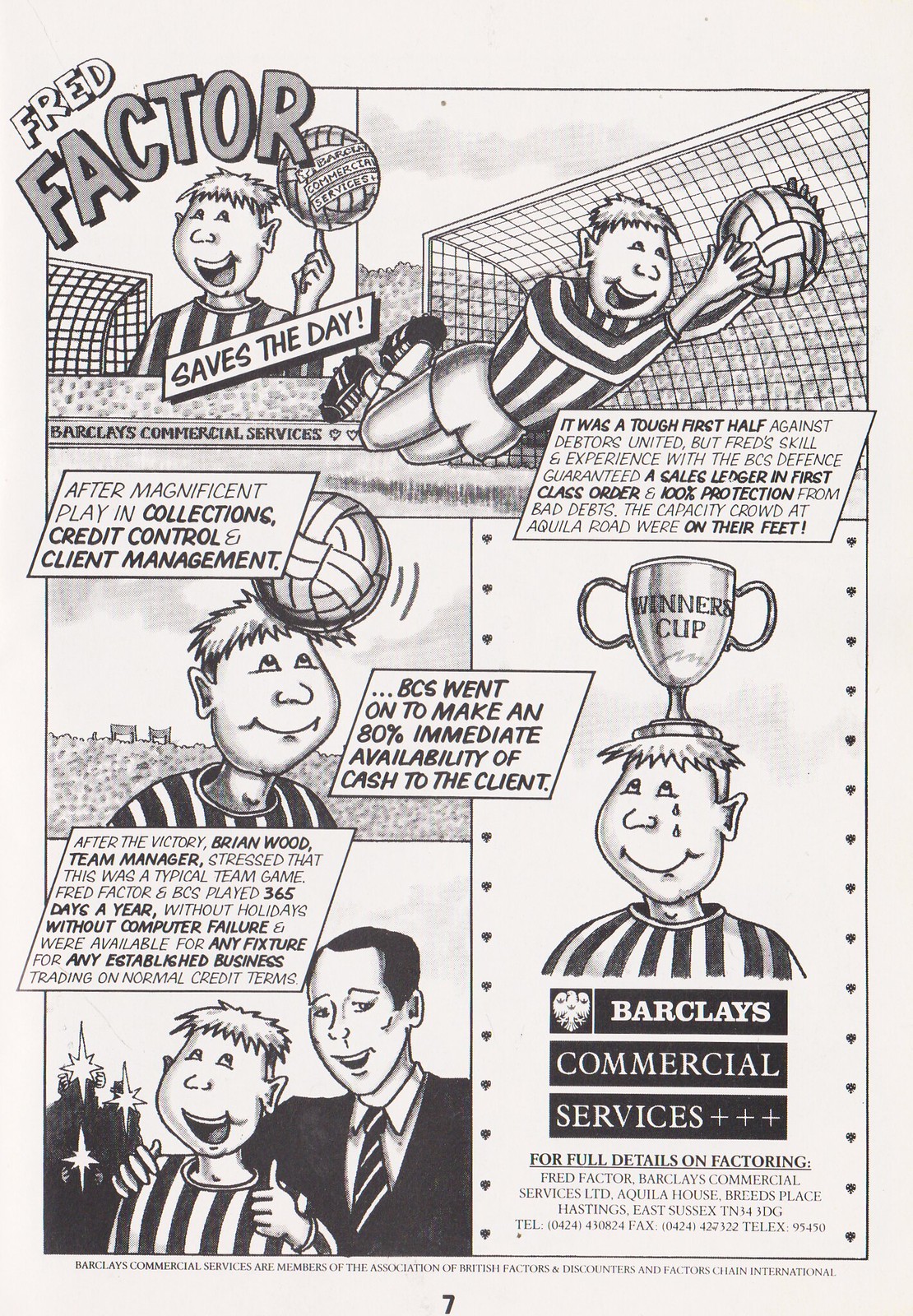In this detailed comic drawing, a boy named Fred Factor, depicted as a heroic soccer player, is the central figure. The comic promotes Barclays Commercial Services through Fred's impressive feats in several frames. 

In the top left frame, under the caption "Saves the Day," Fred is illustrated holding a soccer ball with one finger on his left hand. The top right frame showcases Fred leaping into the air to save a goal, a feat that has the crowd at Aquila Road on their feet. This frame celebrates his skill and experience, which lead to a victorious first half against 'Debtors United.' Moreover, it highlights how Fred’s masterful play in collections, credit control, and client management ensured an 80% immediate availability of cash to the client.

In the bottom right frame, Fred is depicted with teardrops of joy on his face, holding a trophy labeled "Winners Cup" on his head, symbolizing his triumph and the successful services provided by Barclays Commercial Services. The bottom of the comic emphasizes Barclays Commercial Services' reliability and comprehensive credit solutions, boasting 100% protection from bad debts and continuous availability for businesses. Overall, the comic underscores the company’s commitment to financial security and efficiency, illustrated through Fred Factor's celebrated soccer escapades.